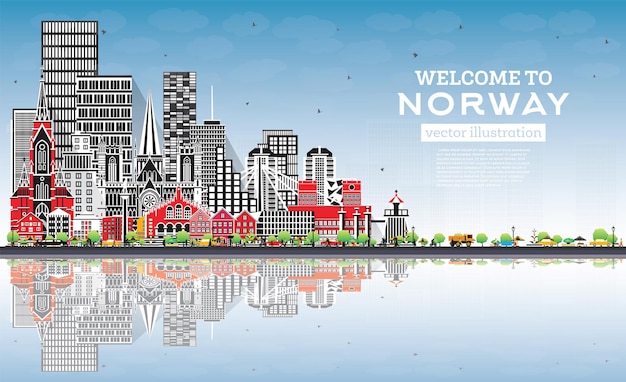The illustration promoting Norway is predominantly blue, transitioning from a vibrant sky to a serene waterfront. On the right side, bold white text declares "Welcome to Norway," with additional reversed white text on blue below it, reading "Vector Illustration," and some tiny, illegible white text beneath. The scene features a cityscape dominated by towering black and white skyscrapers interspersed with a cathedral-like structure marked by a prominent steeple. Closer to the water, a row of red brick buildings, including a large church and a municipal building, enriches the visual contrast. The glassy water impeccably reflects the city's skyline, enhancing the illustration's calm, symmetrical aesthetic. Birds dot the sky, adding life to the tranquil scene. In the foreground, a small yellow vehicle, resembling a dump truck, adds a splash of contrast and detail.